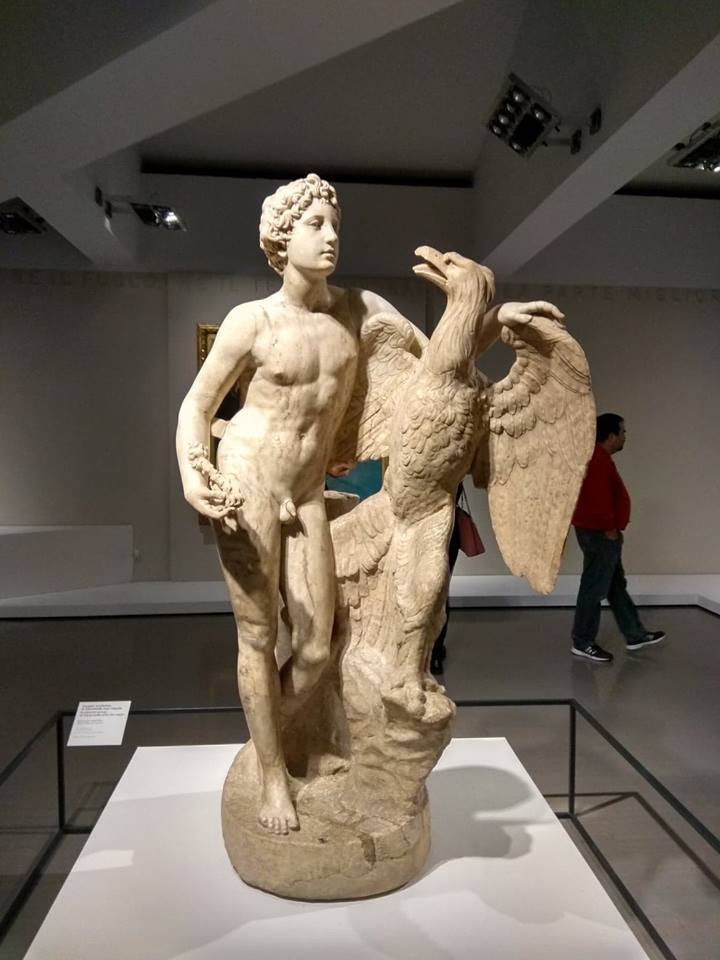The image captures the interior of a museum, focusing on a striking life-size sculpture positioned on a white raised pedestal with a protective metal fence around it. The sculpture, rendered in a tan or golden-brown hue that suggests limestone, depicts a naked young man or teenage boy characterized by his tightly curled, golden-esque hair. He stands beside a grand eagle, almost as tall as he is, with its powerful wings outstretched. The boy appears to be draping his arm around the far wing of the eagle while holding an indistinct object in his other hand at his side. The eagle, with a long neck and prominent beak, gazes intently at the boy's face, while the boy looks past the bird, creating a dynamic interaction between them. In the background, a man in a red shirt and black pants can be seen, adding a sense of scale and context to the scene, along with a few other visitors. There's also a white plaque at the base of the sculpture, although its details are not discernible. Ceiling lights illuminate other exhibits in the gallery, enhancing the museum ambience.